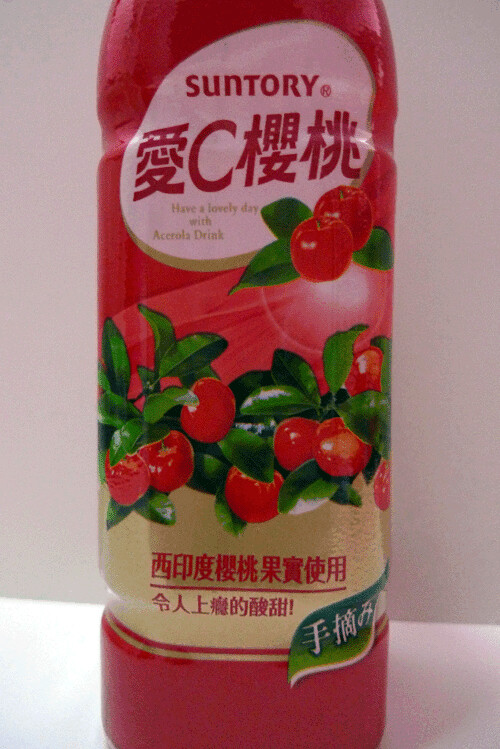A beautifully designed bottle of cherry juice sits prominently against a pristine white surface and matching white wall backdrop. The bottle itself is a vibrant red and made of plastic. At the top, a white oval label bears the brand name "Suntory," followed by Asian characters, most likely Japanese or Chinese. Just beneath these characters, an encouraging message reads, "Have a lovely day with acerola drink." The middle of the bottle features an eye-catching image of ripe cherries flanked by lush green leaves, with two cherries thoughtfully paired and three leaves artistically arranged above them. Adding a touch of elegance, the bottom of the label is adorned with a striking gold band, accented by a subtle green strip encircling the bottle.